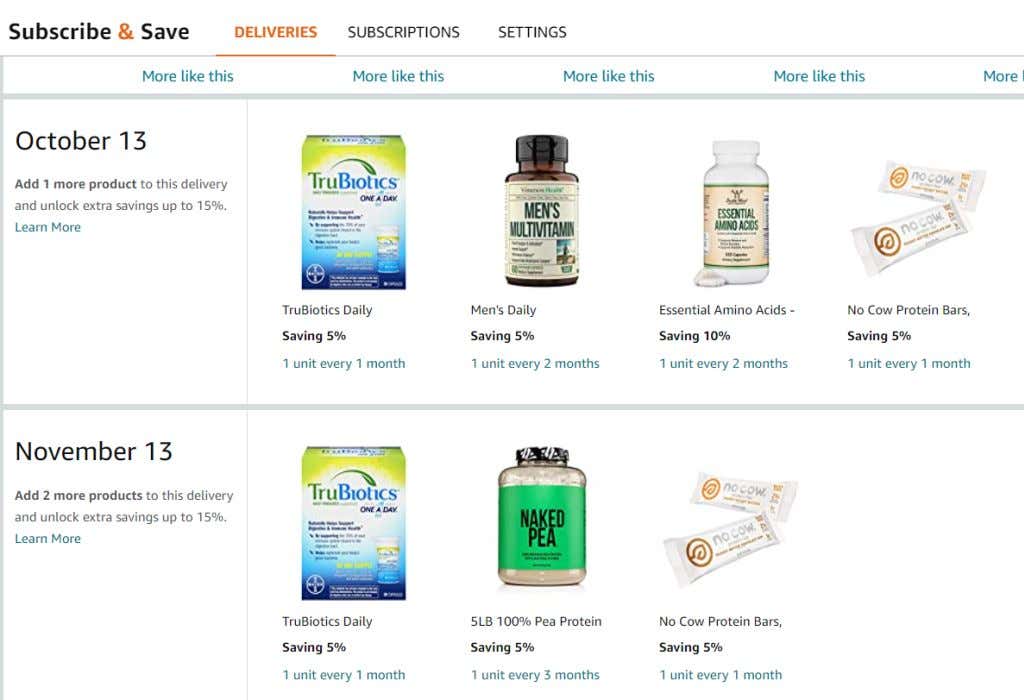This image showcases a "Subscribe & Save" section, possibly from an online retailer like Amazon. At the top, the text "Subscribe & Save" is prominently displayed, with the ampersand (&) symbol in orange while the other words are in black. Below this, the word "Deliveries" is also in orange, followed by "Subscriptions" and "Settings" in black. The topmost section features a repeating banner “More like this” in five places, with the last one partially cut off to just "More."

Moving to the main section, the first row highlights an upcoming delivery scheduled for October 13th, encouraging the user to "Add one more product to this delivery and unlock extra savings up to 15%." A "Learn more" link in blue accompanies this message. The items in this delivery include "True Biotics Daily," "Men's Daily Multivitamin," "Essential Amino Acids," and "No Cow Protein Bars."

Scrolling further down, the next scheduled delivery is for November 13th. Here, the user is prompted to add two more items to achieve a discount. Listed products for this delivery include "True Biotics Daily," "Pea Protein Powder," and "No Cow Protein Bars."

The interface is designed to encourage additional purchases by highlighting potential savings, showing a versatile mix of health and wellness products already in the user's subscription list.